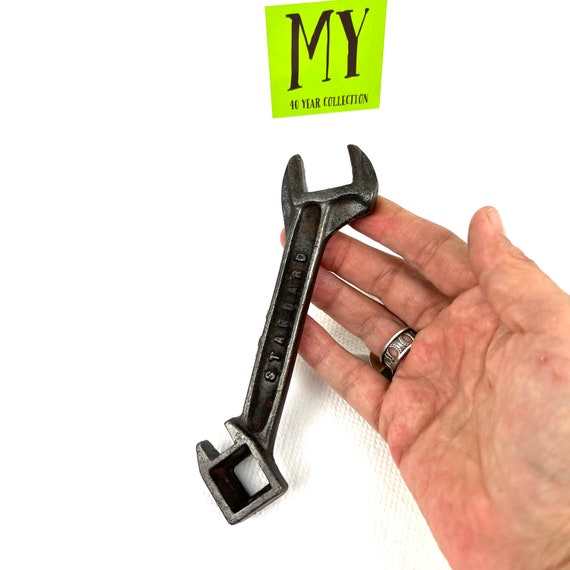In this photograph set against a white background, a man's right hand, palm-up, is prominently displayed, with a focus on his ornate silver wedding band with intricate cutouts adorning his ring finger. Resting delicately on his fingertips is an unusual and antique wrench. This wrench features a conventional open-end at one end and a unique square end with small, stationary points that resemble calipers at the opposite end. The handle of the wrench is inscribed with what appears to be "Starbird" or a similar name. Above the man’s hand, there is a lime green, flat square illustration that is hand-lettered with the phrase "MY 40-YEAR COLLECTION" in bold black letters, indicating that the wrench is part of a long-held personal collection.